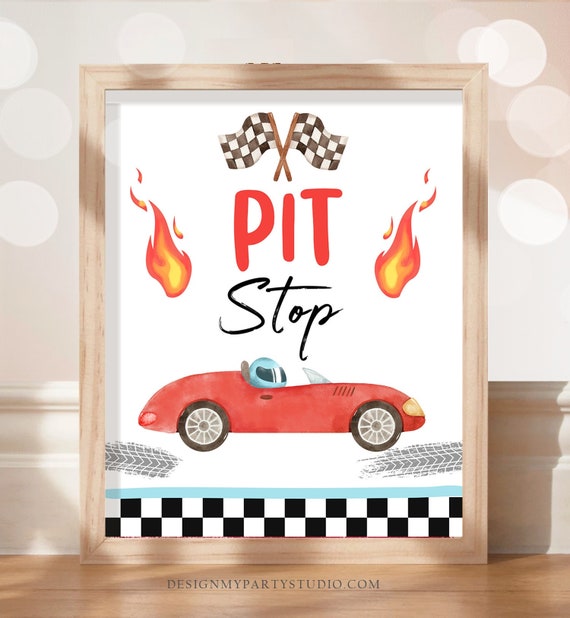The image features a detailed and vibrant poster set against a light-colored hardwood floor and a white wall. The poster, enclosed in a wooden frame, prominently displays the words "PIT STOP" at the top. "PIT" is written in bold red capital letters, while "STOP" is in black. Above the text, two checkered flags cross each other in the top center of the poster. On either side of the word "PIT," small flames add a fiery touch. Below the text, a vividly illustrated red race car with black tires is depicted, driven by a figure wearing a blue helmet with a visor. The car is positioned facing right, with tire skid marks underneath indicating movement. These skids are flanked by blue stripes, followed by light blue and black-and-white checkered patterns at the bottom. Resting on the floor, the poster includes the website address "designmypartystudio.com." Light from the left side of the image casts subtle reflections on the floor, enhancing the picture's dynamic feel.